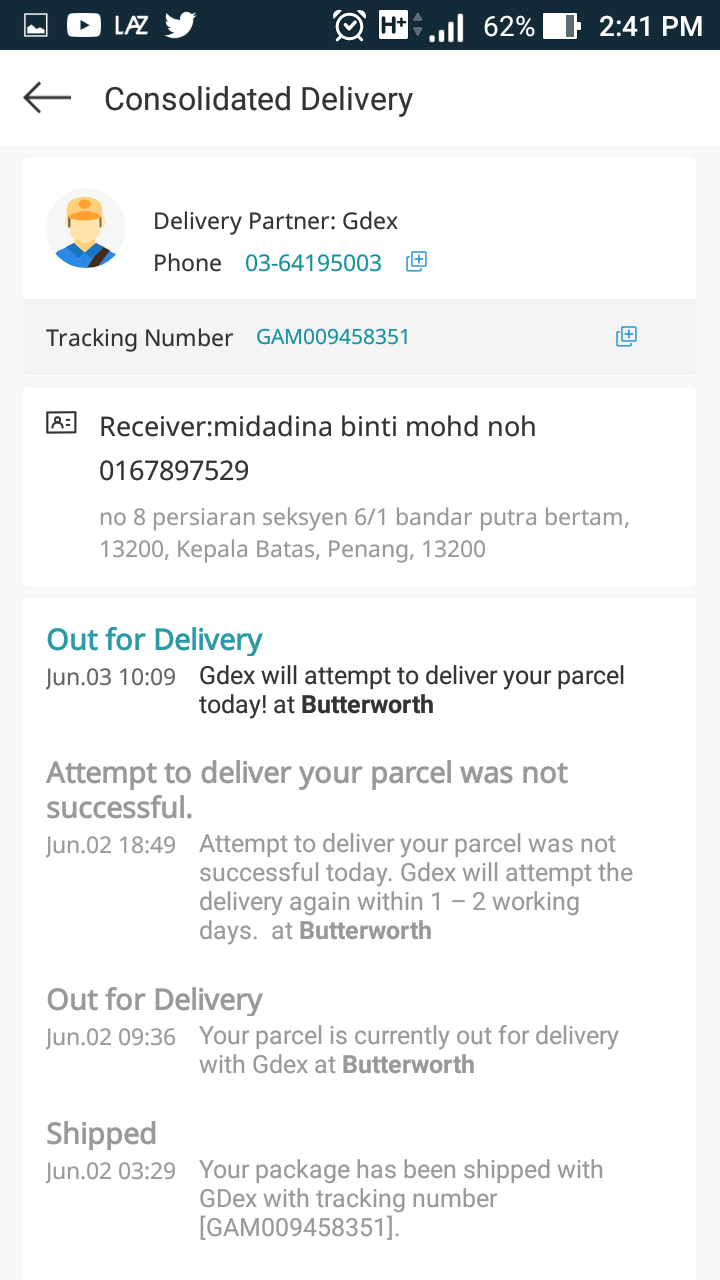### Detailed Caption for a Cell Phone Screenshot

The screenshot captures a detailed delivery tracking screen with a white background. A black bar at the top displays various icons from left to right: a photo icon, a video icon, the LAZ app icon, a Twitter tweet icon, an analog clock icon, a "H+" symbol (indicating mobile data type), a signal bar icon showing connection strength, a "62%" battery percentage, and finally a battery icon. On the far-right corner, it displays the current time: 2:41 PM.

Directly below the black bar, the heading reads "Consolidated Delivery" accompanied by a back arrow pointing to the left. Below this heading, there is a circular icon representing a delivery partner—a faceless Caucasian man wearing a blue shirt and yellow hat. To the right of the icon, the text states "Delivery Partner: GDX Phone" followed by the contact number in blue text: "03-641-95003."

The next section lists detailed tracking information. In black text, it reads "Tracking Number," and next to it in blue text is "GAM009458351." Further down, "Receiver:" is followed by "Mid and Dina Binti Mod No.," and below that is a contact number, "016-789-7529."

Address details are listed as follows: "No. 8, Persiaran, 6 in 6 out of 1, Bandar Putra Bertam, 13200, Kepala Batas Penang, 13200." In blue text, the status updates to "Out for Delivery."

The chronological tracking history is as follows:
- **June 3rd, 10:09 AM:** The black text indicates, "GDX will attempt to deliver your parcel today at Butterworth."
- **June 2, 18:49 PM:** The delivery attempt was not successful. A message notes, "Attempt to deliver your parcel was not successful today. GDX will attempt the delivery again within 1-2 working days at Butterworth."
- **June 2, 09:36 AM:** Text updates, "Your parcel is currently out for delivery with GDX at Butterworth."
- **Shipped June 2, 03:29 AM:** The final update is about the shipment confirmation, "Your package has been shipped with GDX with tracking number GAM009458351."

This comprehensive caption offers a clear, step-by-step tracking process and relevant information for the package delivery.